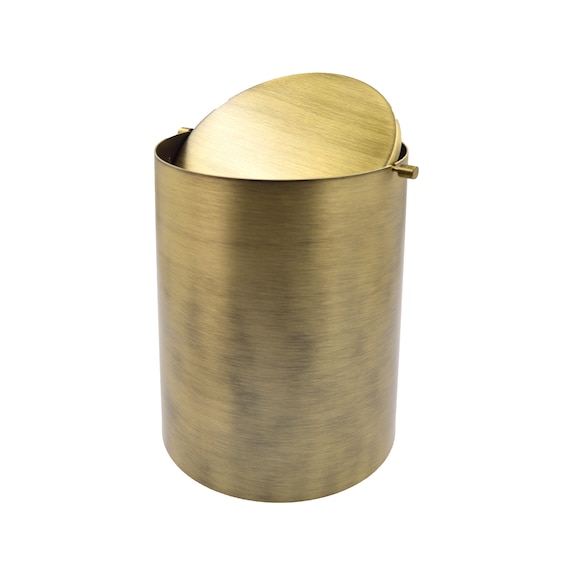This image showcases a large, cylindrical container that appears to be a burnished metal, possibly an alloy of copper and brass, giving it a brushed appearance. The container is prominently set against a white background to highlight its features. It's constructed from wood but finished to look like metal, displaying distinct circular striations that suggest it has been sanded down. The vessel includes a lid equipped with a swiveling mechanism, akin to a butterfly valve, mounted on two knobs on either end of a metal rod. This mechanism allows the lid to pivot, enabling access from either the left or right side. The overall design hints that it could function as a trash or compost bin, given its size and shape, reminiscent of a five-gallon container.